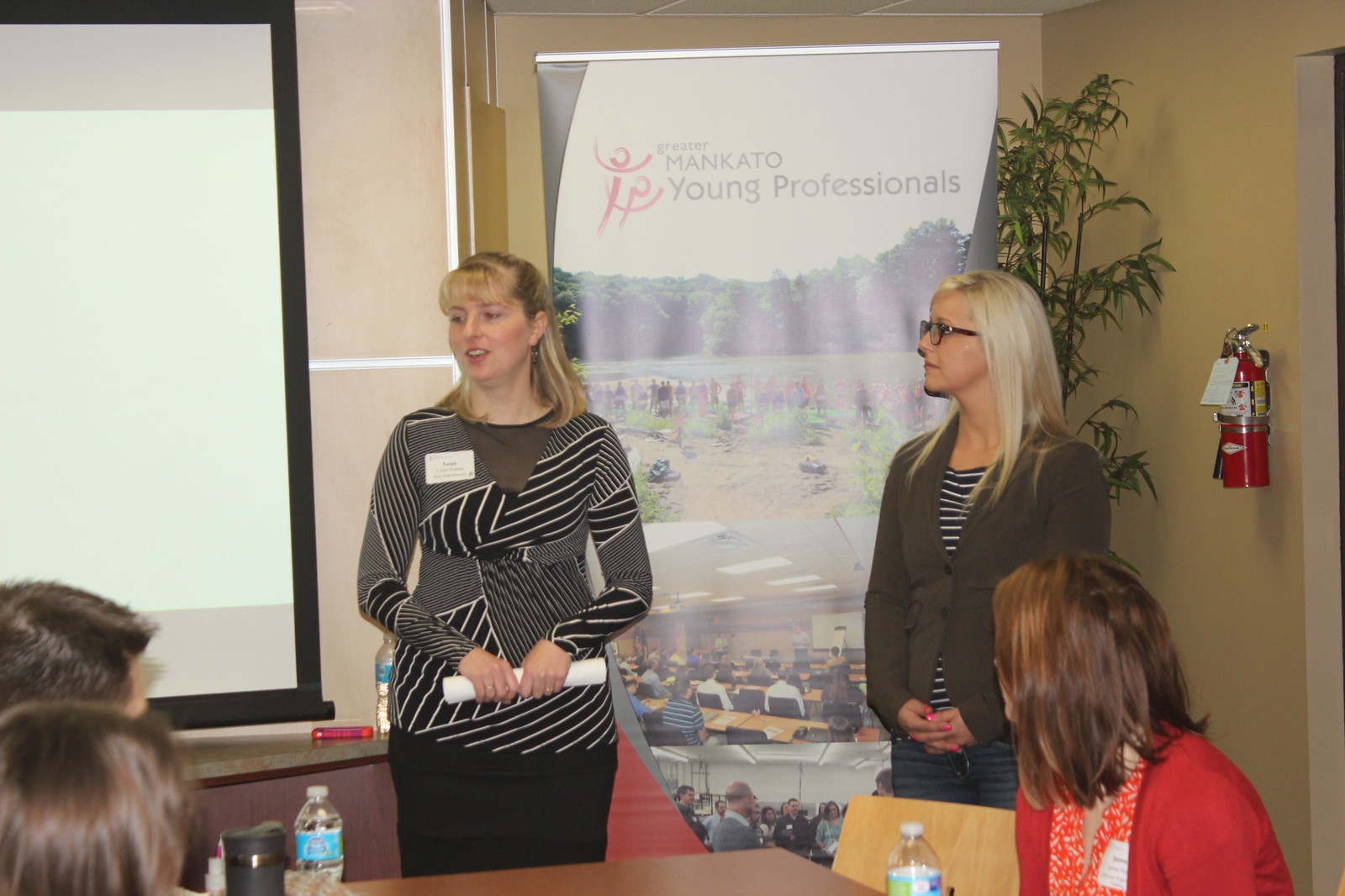The image features two women standing in front of a freestanding poster banner that reads "Greater Mankato Young Professionals." The woman on the left is wearing a black and white abstract striped top with various lines of different thicknesses, paired with a black skirt. She has blonde hair, a white badge on her chest, and is holding a rolled-up piece of paper with the back of her hands facing outwards. She gazes downward to the bottom left of the image, with her mouth slightly open. The woman on the right is dressed in a light-gray jacket over a black and white t-shirt and is wearing glasses. With blonde hair and a neutral expression, she looks off to the left side, her hands cupped together in front of her waist. 

In the foreground, two individuals can be seen at the bottom left of the image, seated at a table adorned with coffee cups and water bottles. These people appear to be attendees of the event, dressed in business attire, indicative of a conference or presentation setting. Behind the women, the poster features red outlines of two figures, an outdoor group photo, a classroom scene, and another group image running vertically.

The scene is set in an indoor office or building space, indicated by the presence of a projector screen on the left and a fire extinguisher and door on the right. The overall atmosphere suggests that the women are involved in presenting or recruiting for the Greater Mankato Young Professionals organization.